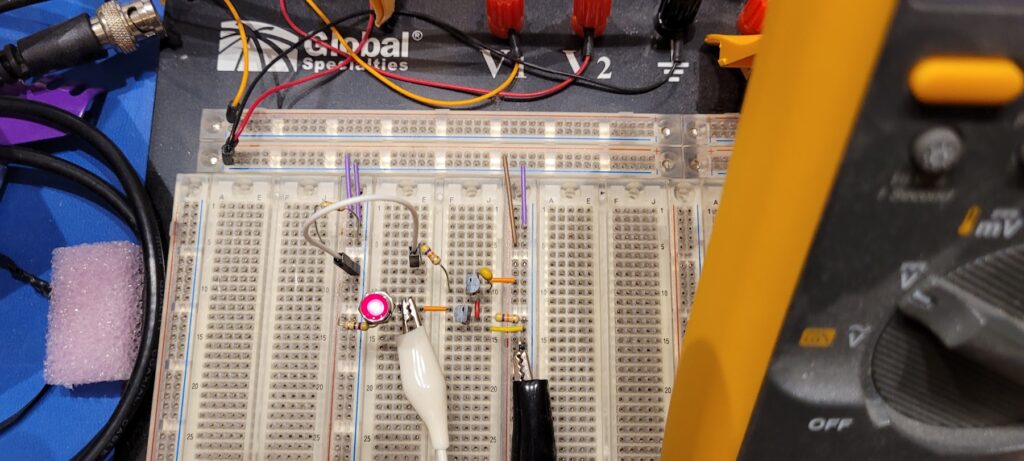The image depicts a top-angle view of a complex electronic setup, likely a component of a science kit or educational equipment for working with electrical circuits. The centerpiece is a white patch board with numerous square peg holes, where various resistors and wires are connected. Several wires of different colors—black, red, yellow, and white—are attached to different points on the board. Notably, there are black and white clamps, presumably connecting to a multimeter partially visible on the right-hand side of the image, featuring a yellow side and a black dial. Above the patch board, there is a black box labeled "Global Specialties" with V1 and V2 markings, alongside red, black, and yellow twist caps. Additional components include a black circular jack, a piece of sponge, and assorted knobs and switches, hinting at a more extensive setup for electrical experimentation or learning.